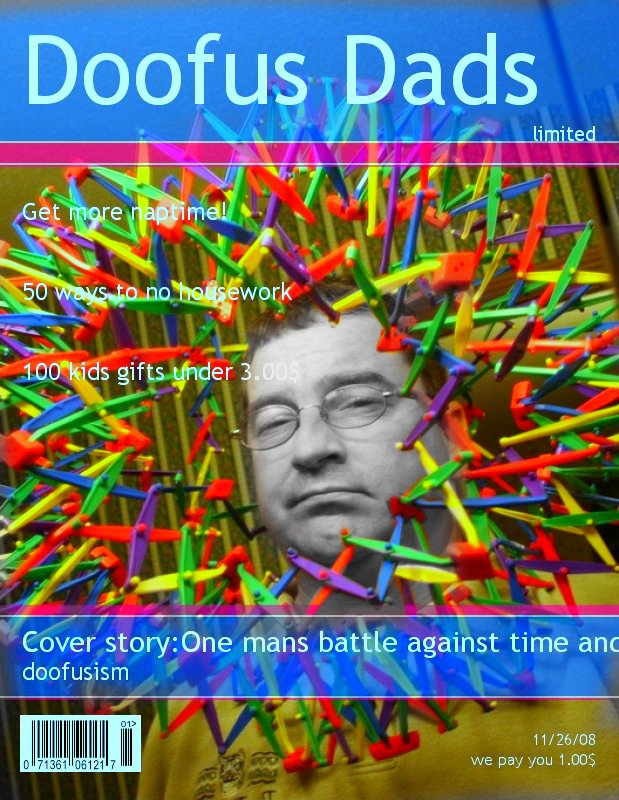The magazine cover features a portrait of a man wearing wire-rimmed glasses and a yellow polo shirt, partially concealed by a sweater with a detail on the right chest. Encircling his head is an expanded collapsible rainbow-hued toy made of interlocking sticks and gears, reminiscent of a childhood toy that can be compressed into a tight ball. The top of the cover features the heading "Doofus Dads" in white text on a light blue background, with the word "Limited" underneath to the right. Just below, there is a pink horizontal stripe. Near the base of the cover, a blue band contains white text that reads, "Cover Story: One Man's Battle Against Time and Doofusism." The bottom left corner bears a barcode with the numbers 071361061217, while the bottom right corner displays the date 11-26-08 and the text, "We pay you $1."